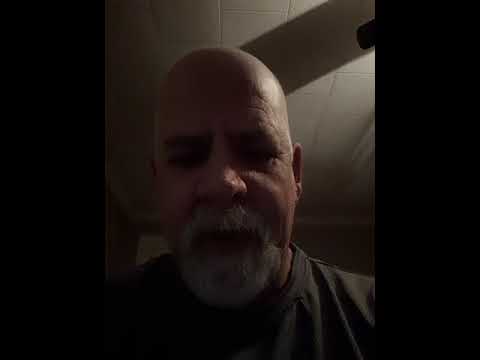The photograph depicts an older Caucasian man with a bald head and a mostly white goatee, consisting of a beard covering his chin and a mustache above his lips. His face shows signs of age, with visible lines around his eyes. The man is wearing a dark-colored shirt, possibly green or black, which appears somewhat raggedy. He is taking the photograph himself, likely a selfie, as he looks somewhat downward into the camera. The setting is a dimly lit cellar-like room with numerous shadows, making it difficult to discern all the details in the background. The ceiling behind him consists of white box tiles, and there is a partially closed door that suggests the light source is off to the right. Thick black bars frame the left and right sides of the image, which are not part of the photograph but are noticeable in the image's composition.